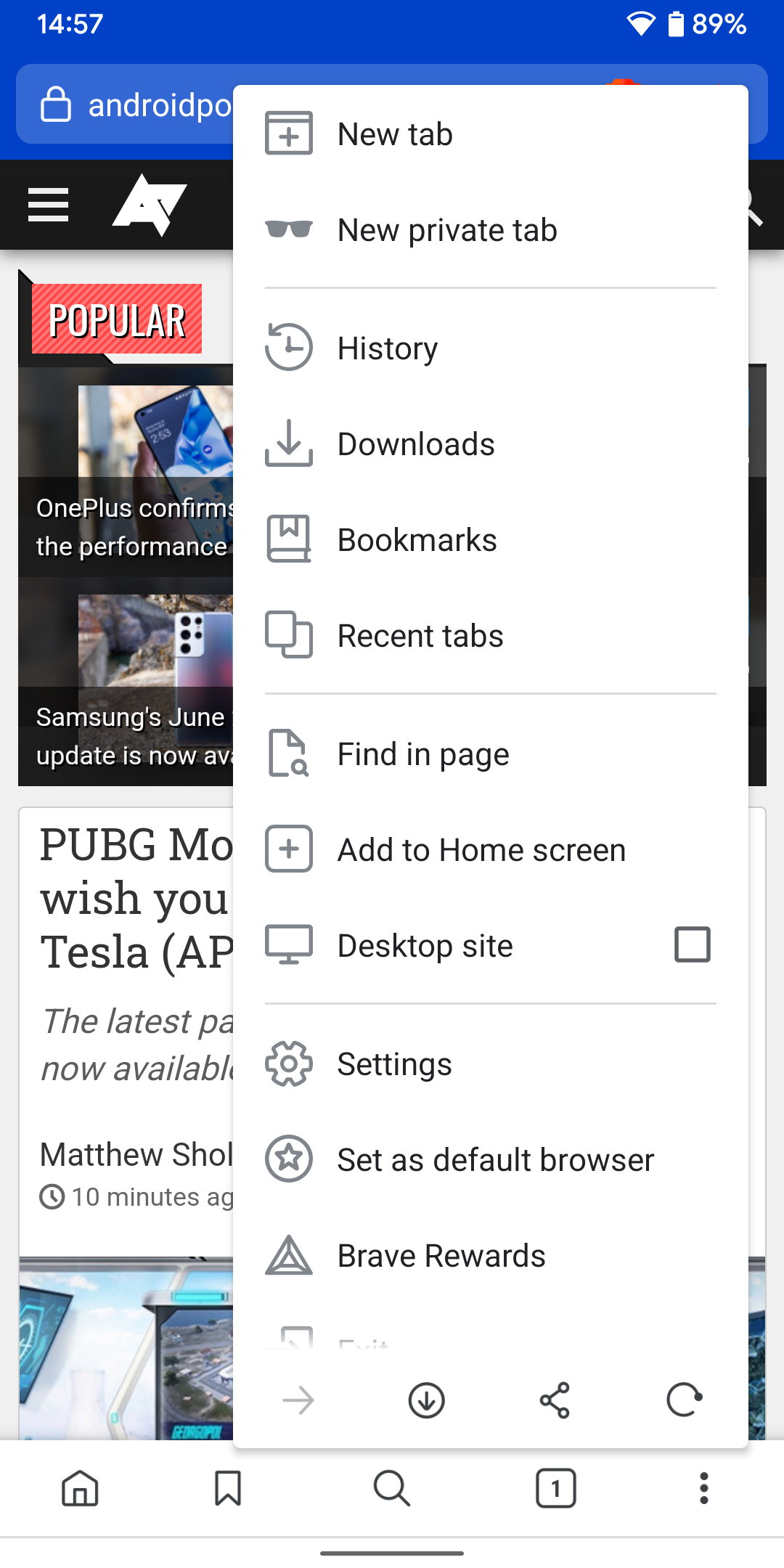The image is a screenshot from a cell phone. At the top, there is a blue header with white text. In the upper left corner, it shows the time as 14:57, while the upper right corner displays icons for Wi-Fi and a battery level at 89%. Below the header is an open white box containing a menu. This menu features a series of options in dark gray text against a light gray background.

The first option is "New Tab," followed by "New Private Tab," which includes an icon of dark sunglasses to its left. Below these options is a light gray horizontal line. The menu continues with options labeled "History," "Downloads," "Bookmarks," and "Recent Tabs," followed by another horizontal light gray line.

Further down, the options "Find in Page," "Add to Home Screen," and "Desktop Site" are listed, separated by another horizontal line. At the bottom of the menu are the options "Settings," which includes a settings icon, "Set as Default Browser," and "Brave Rewards."